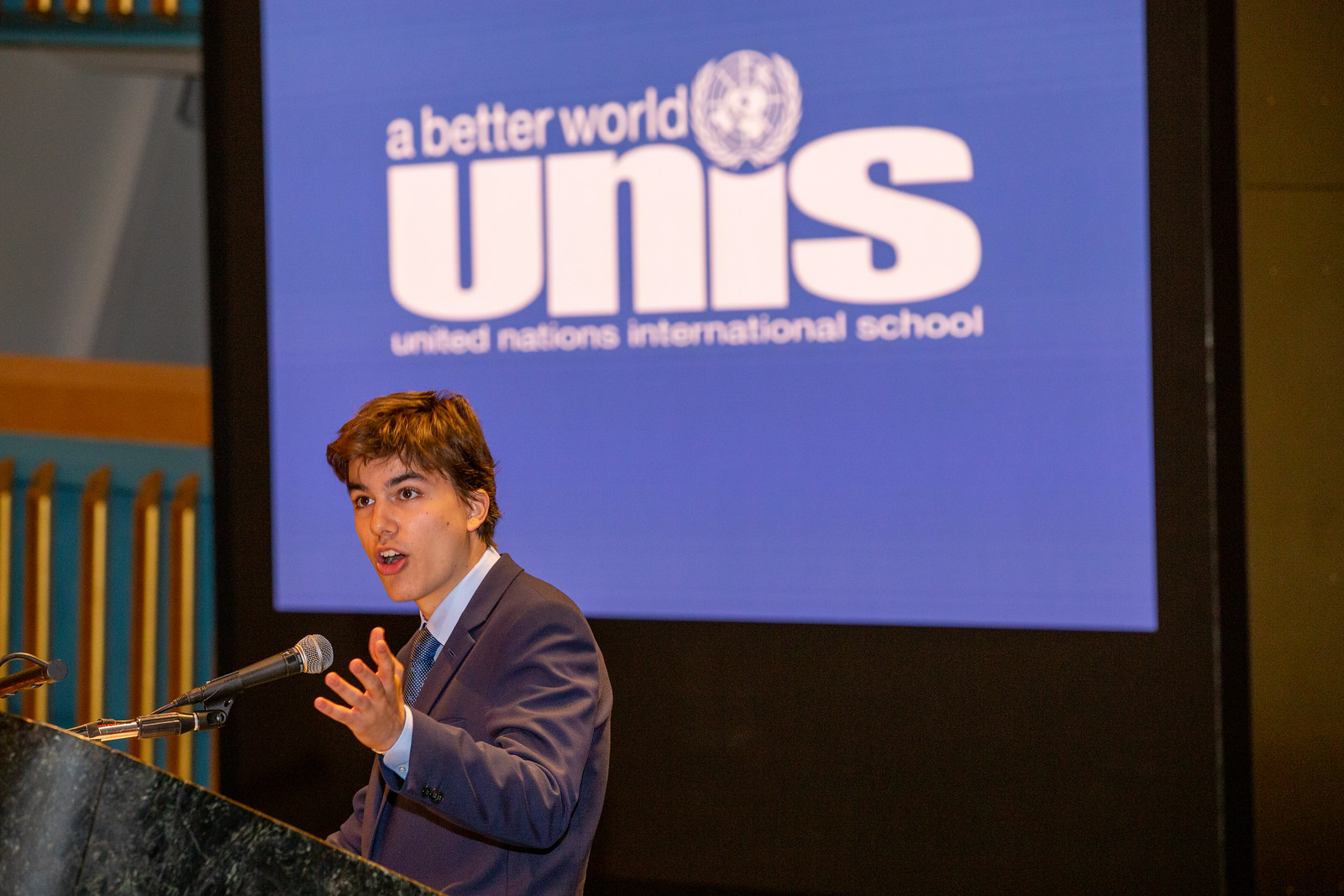In the image, a young man, dressed in a gray suit, light blue shirt, and dark blue tie, is speaking animatedly from behind a black and gray marble podium, his left hand gesturing upward. A microphone extends toward his mouth, which is slightly open as he looks straight ahead. His short brown hair is neatly styled. Directly behind him, a large blue screen displays the text, "A Better World UNIS, United Nations International School," with the "I" in "UNIS" stylized as a globe. The background is primarily gray, accented by a teal section on the left wall adorned with at least five gold-colored bars. The scene appears to be set indoors during a conference or presentation, with emphasis on the young man at the podium as the central focus.